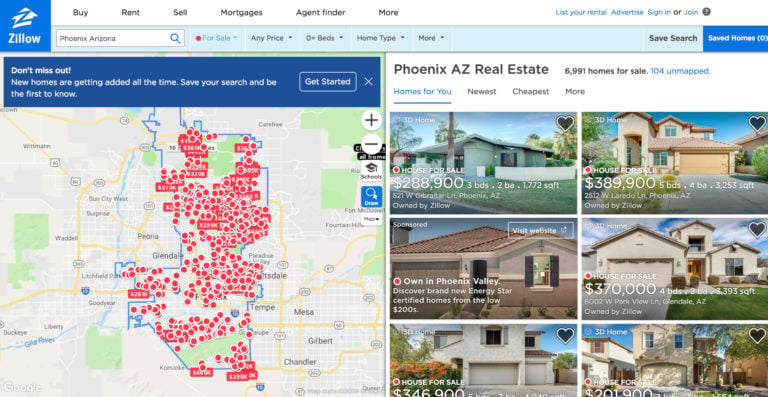This is a detailed and descriptive caption for the given image:

---

This screenshot from Zillow's website prominently displays the Zillow logo in the upper left corner. Running across the top of the screen is a navigation bar with the options: Buy, Rent, Sell, Mortgages, Agent Finder, and More. Below this, there's a search box where the text "Phoenix, Arizona" is entered. Next to the search box, a "For Sale" option is highlighted in blue, bearing a red dot next to it.

Beneath the search bar, a map spans the area, and above this map is a header that reads: "Don't miss out. New homes are getting added all the time. Save your search and be the first to know." The map itself is dotted with numerous overlapping red dots, representing available properties, and features some partially legible text indicating various locations such as Surprise, Waddell, Glendale, Mesa, Gilbert, Tempe, Liberty, and Buckeye. Scattered on the map are a few red rectangles with blurry, hard-to-read prices in them.

To the right of the map, the screen showcases photos of six homes available for sale. At the very top is a header stating: "Phoenix, Arizona real estate, 6,991 homes for sale," with "Homes for You" highlighted in blue. Each home listing includes an exterior shot of the property along with detailed information such as the price, number of bedrooms and bathrooms, and the square footage. Additionally, in the upper right corner of each photo, there's a black-filled heart icon, indicating the homes have been favorited.

---